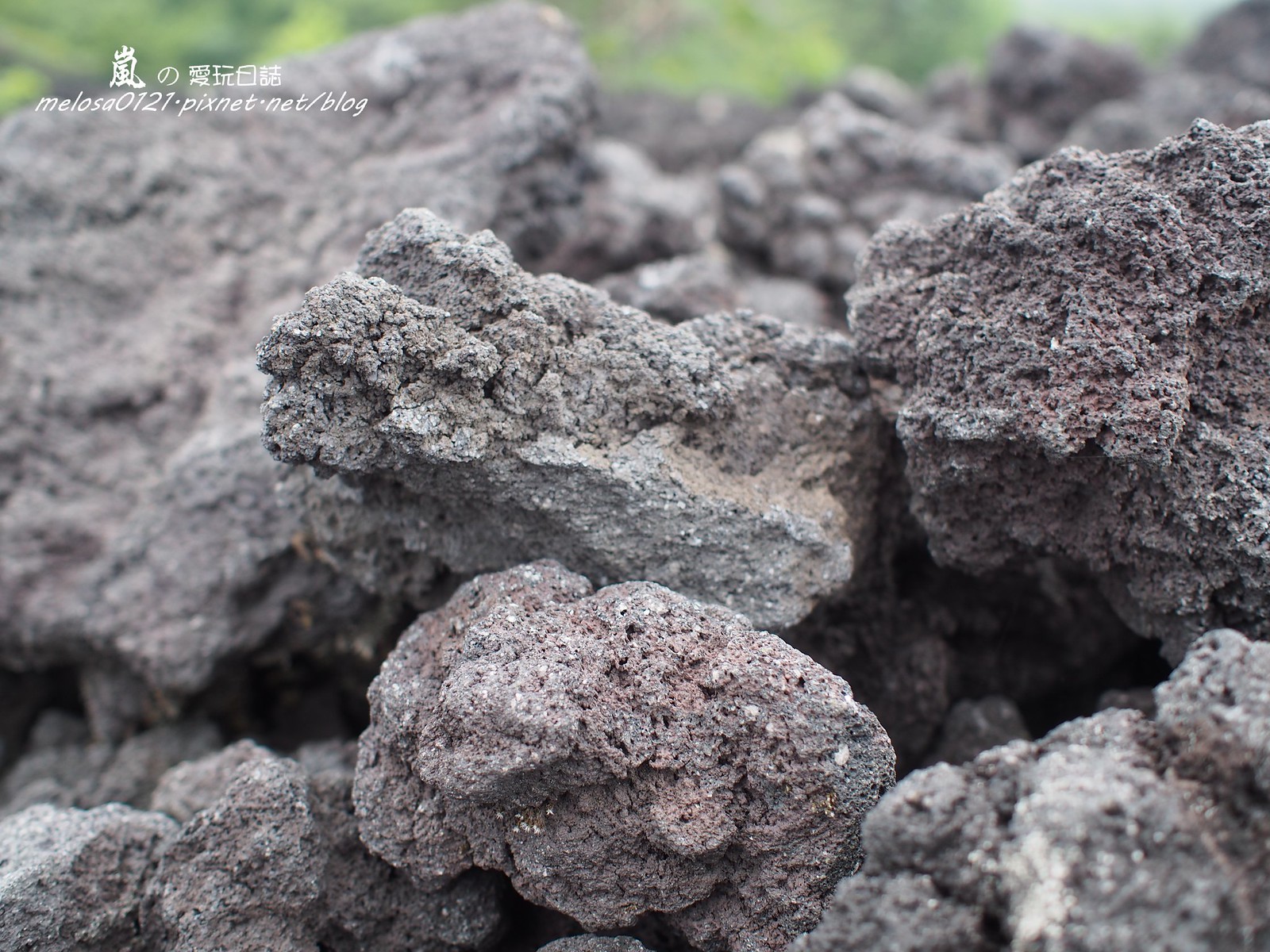The photograph captures a detailed close-up of a pile of gray rocks, possibly including lava or cement rocks, with smaller broken stones stacked on top of each other. Amidst the slate gray rocks, there are shadings of purple, maroon, beige, and white. The high-definition image reveals intricate details such as the pores and textures of the rocks. In the background, slightly out of focus, stretches greenery consisting of various shades of green, suggesting the presence of trees, bushes, or grass. At the top left corner, there is text in an Asian script, possibly Chinese or Japanese, followed by "melosa0121pixnet.net/blog" in white italic letters. The photograph appears to be taken outdoors, likely during daylight hours, offering a stark contrast between the sharp details of the rocks in the foreground and the blurred vegetation behind.